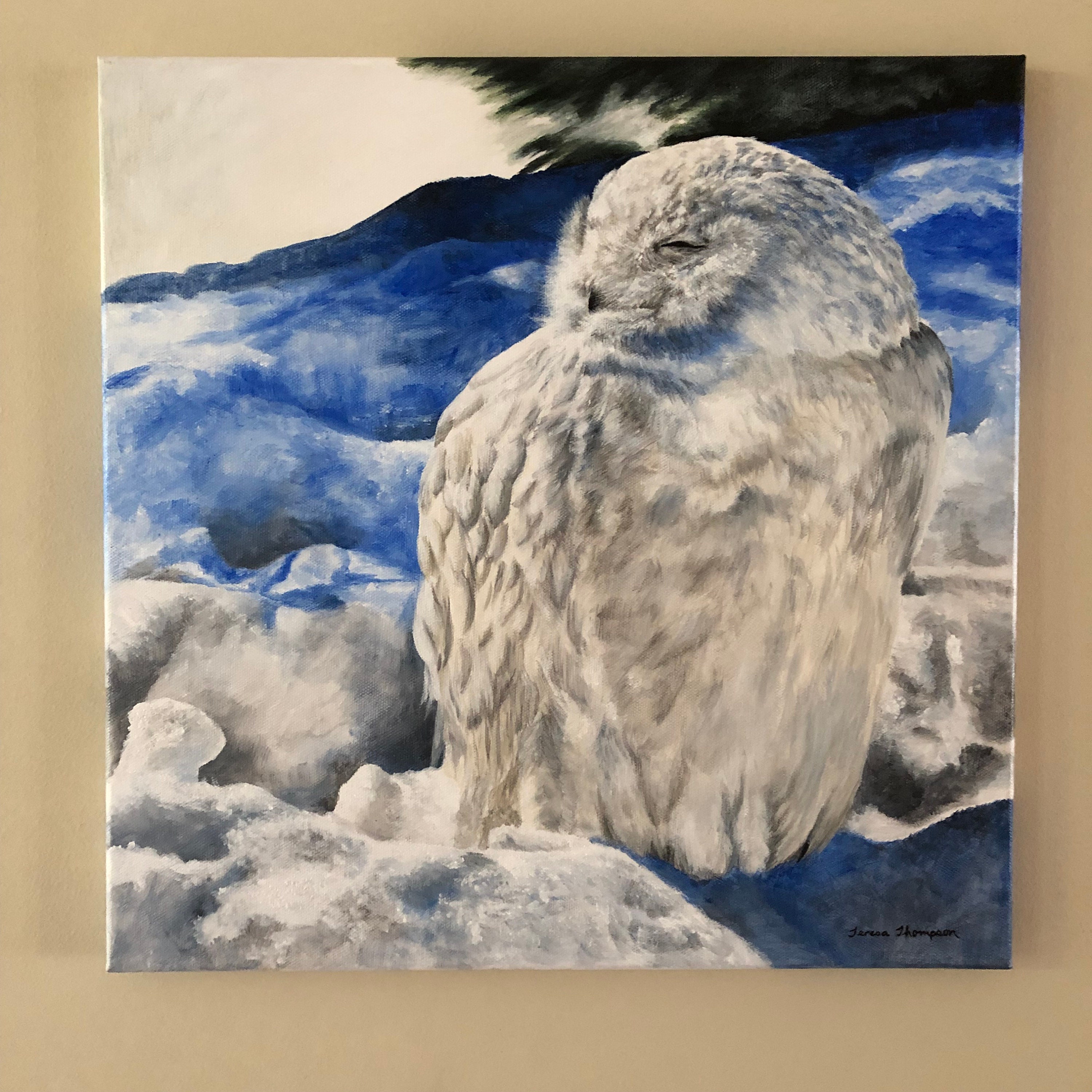This detailed photograph showcases a striking piece of wall art mounted on a beige wall. The artwork, which is square in shape, vividly depicts a large, fluffy-feathered grey owl, meticulously painted to highlight its white and black coloration. The owl, with its head turned and eyes partially open, gazes to the left, perched atop a greyish rock rather than a tree branch. The backdrop features a serene, tanny white sky with a silhouetted tree rendered in dark hues in the top right corner. Blue-toned mountains, suggesting a snowy landscape, provide a contrasting background that subtly enhances the owl's distinct coloration. This intricate painting, seemingly executed in watercolors, bears the artist’s signature in black ink at the bottom right corner. The entire piece is framed in a beige-tan border, adding a sophisticated touch to the artwork.